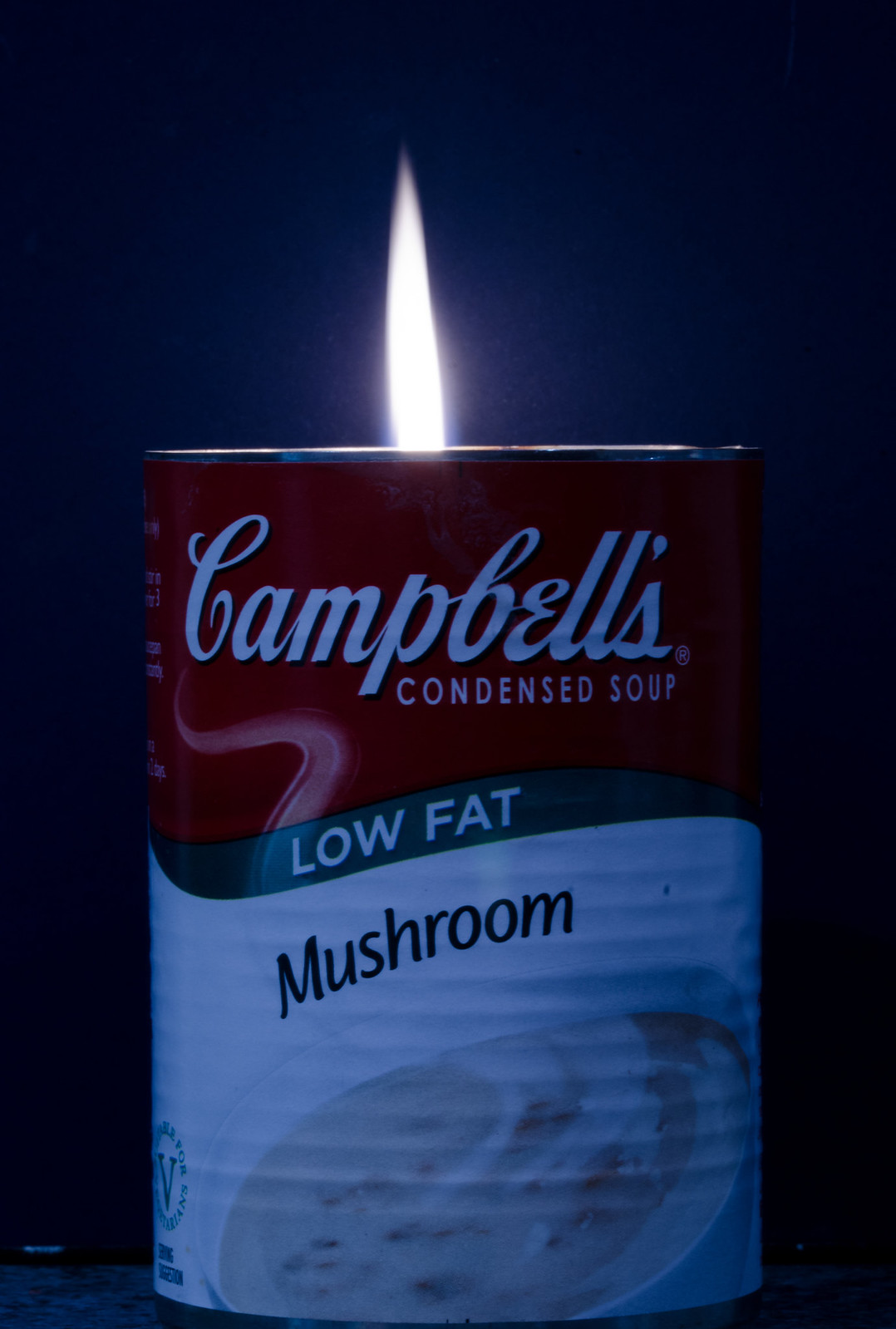In this pop art-inspired image reminiscent of classic clip art, we see a tin can distinctly labeled as "Campbell's Condensed Soup." The word "Campbell's" is elegantly inscribed in white cursive text, with "Condensed Soup" appearing in smaller text beneath it. The can's upper half features a vivid red background, which prominently displays the Campbell's logo, while the lower half transitions to white, offering a textured visual experience.

The can's label showcases a green ribbon-like shape with "LOW-FAT" written in bold, all-caps letters. Below this ribbon, in black text, is the word "Mushroom," specifying the soup variety. Additionally, an illustration of a creamy bowl of mushroom soup, characterized by its light gray color and dotted with tiny chunks of mushrooms, captures the viewer’s attention.

Emanating from the center of the can's top is a striking element—a white flame, about three inches tall and half an inch wide, giving the can an almost surreal, luminous quality. This flame seems to emit light, contributing to the overall blue tint of the image. The backdrop is a dark blue wall, creating a dim, almost moody atmosphere. The can itself rests upon a dark-colored table, further enhancing the image’s depth and richness in this evocative pop art setting.